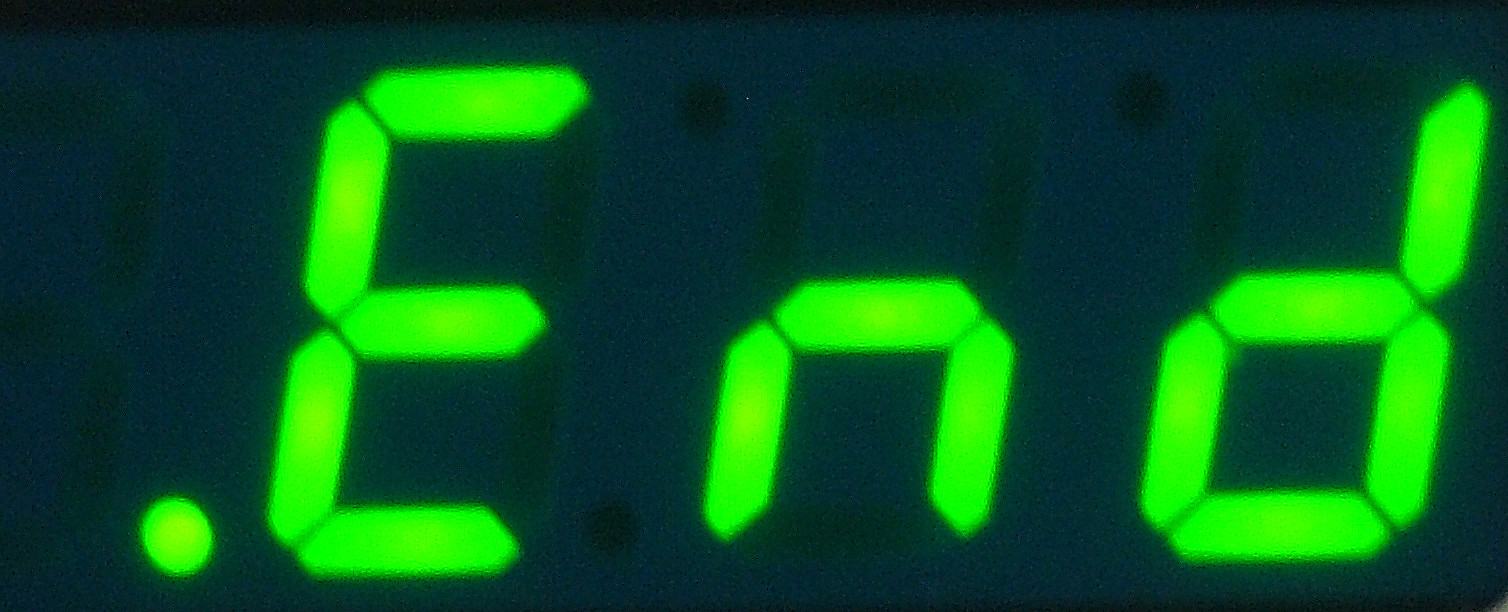The slightly blurry photograph captures a digital display likely from a microwave. The display features the word "END" in a neon lime green font, preceded by a dot (period). The characters, reminiscent of digitized numbers found on an alarm clock, are formed by segmented portions and appear blurry themselves. The background of the image is a bluish-black, revealing ghosted remnants of previous numbers due to a burn-in effect. Surrounding the display is a faint black border and a small white sliver at the bottom on one side. The image is slightly pixelated, adding to its overall blur. There are no other elements present in the image, allowing the illuminated green "END" to dominate the space.